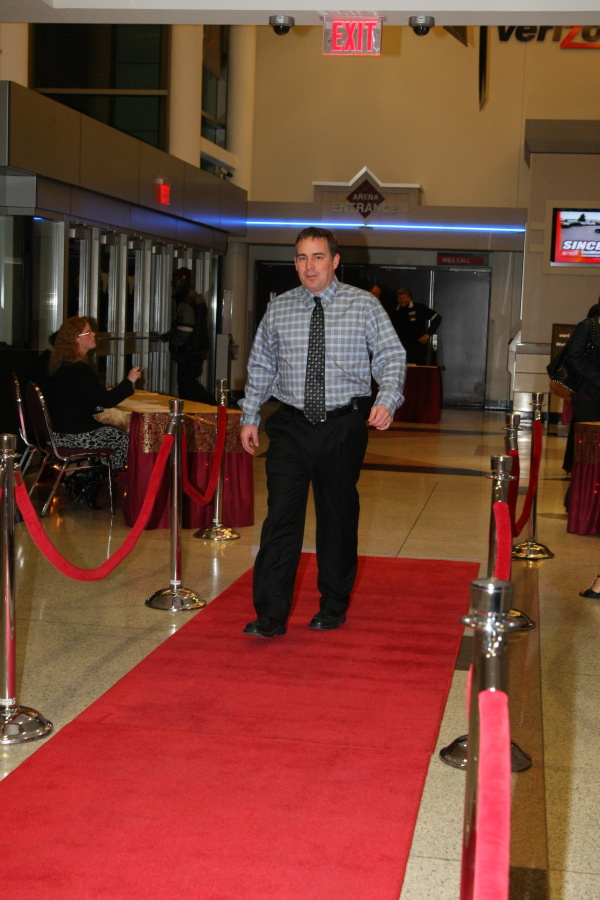This indoor photograph captures a man in the center, striding purposefully on a red carpet bordered by velvet ropes on both sides. The carpet lays atop a smooth, light brown, glossy floor, suggestive of a convention center setting. The man sports a blue and white checkered long-sleeve shirt, paired with black pants, black shoes, and a black tie accented with white polka dots. His arms swing slightly at his sides, indicative of a natural walking motion. 

To his right, a woman with red hair, clad in a black shirt and a black and white skirt, sits at a table, possibly awaiting to sign people in for the event. The left side of the image shows an exit sign above additional doorways. Directly behind the man, signage for an arena entrance is visible, along with several individuals, including what appear to be security personnel positioned before a monitor and additional tables with people standing behind them. At the upper section of the photograph, "Verizon" is printed in dark letters against a yellow wall, above an inset computer screen. This vibrant setting is bustling, but the focus remains squarely on the man walking forward on the red carpet.